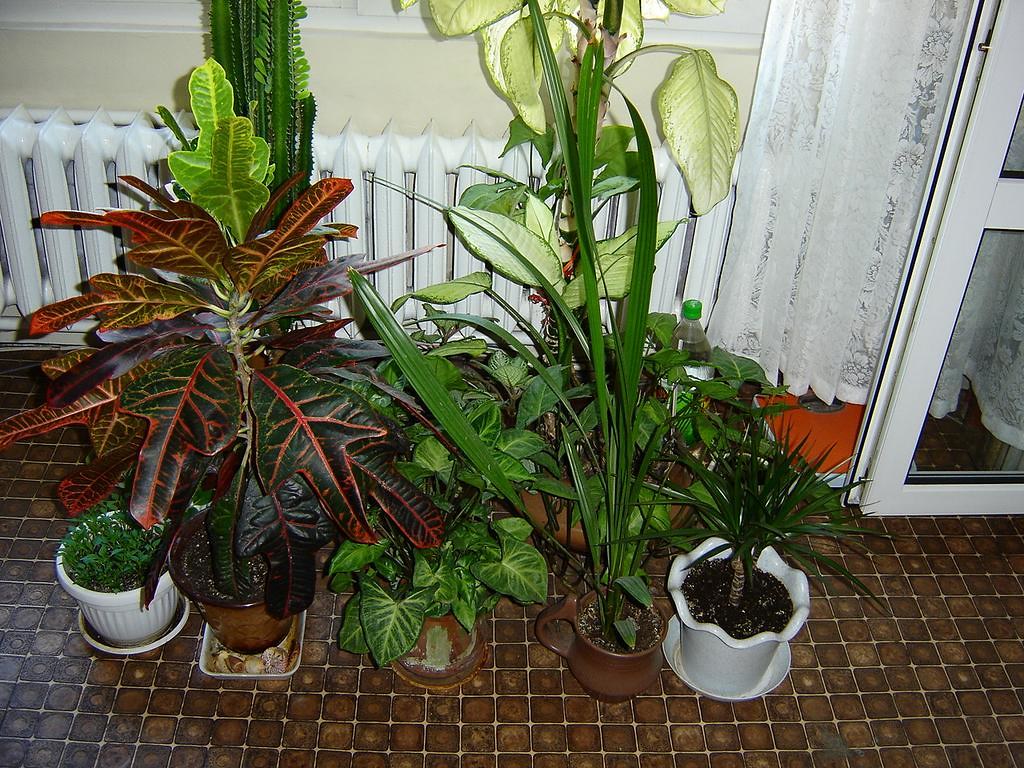This indoor photograph showcases five potted houseplants arranged on a floor with a distinctive checkered brown pattern that resembles copper pennies, accentuated by white grout. In the background, there’s an old-fashioned white radiator vent against an off-white wall, with a lace curtain partially visible near a see-through glass door. The plants, nestled closely together, offer a diverse display of greenery. On the far right, a spiky plant sits in a white pot. Next to it, a single tall green-leafed plant grows from a coffee cup. A lush ivy occupies a brown pot beside it, followed by a rubber plant also in a brown pot. The assortment is rounded off by a very short, cropped plant in a white pot. The variations in plant types and pot colors enhance the picturesque indoor setting.